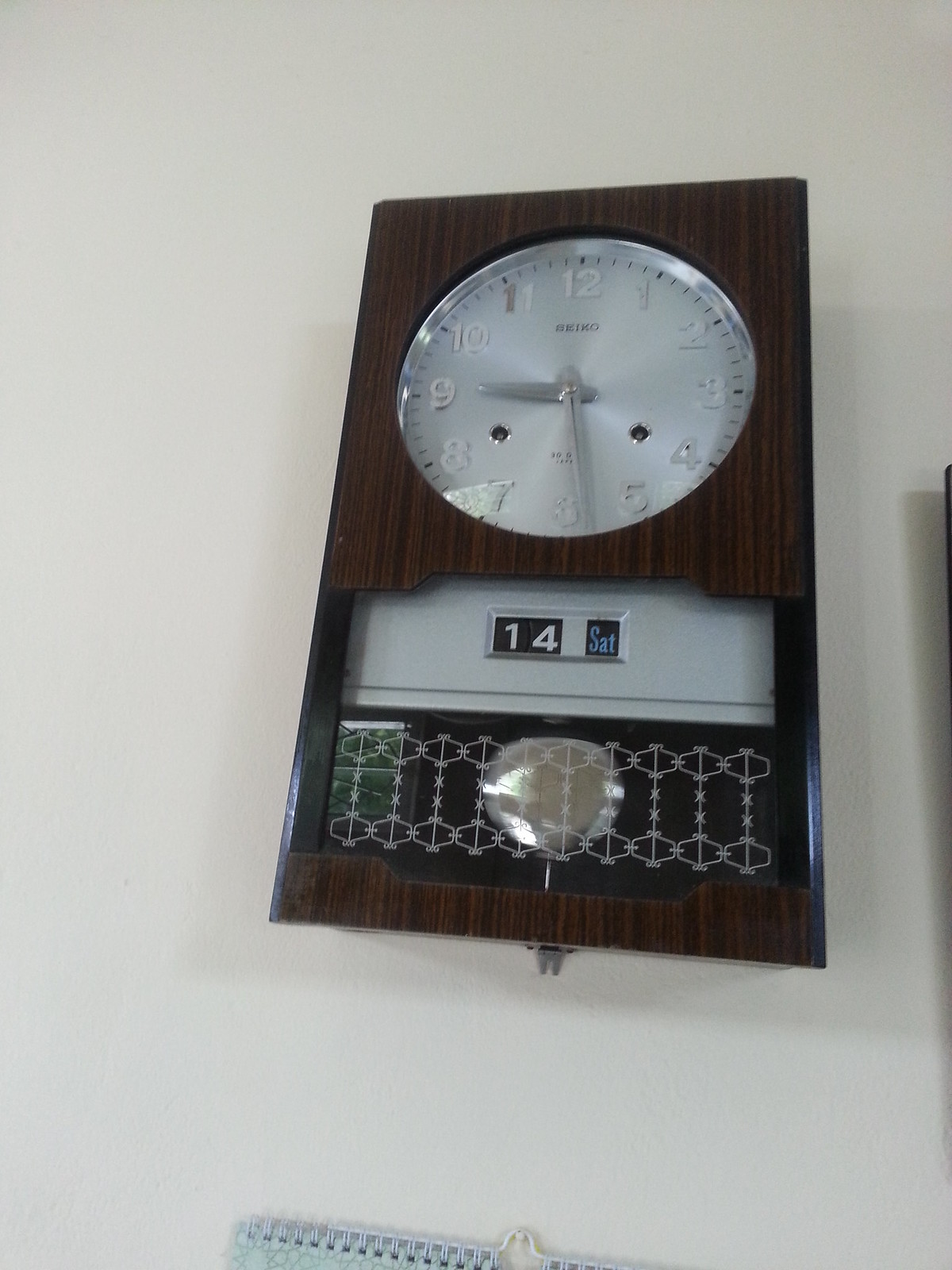This image showcases a modern wall-hanging clock inspired by traditional grandfather clock design. It features a sleek, rectangular case crafted from dark cherry wood, exuding an elegant and timeless appeal. The upper section of the clock displays a large, round silver face with white numerals encircling it. The time indicated is 9:29, with the hour and minute hands also in silver. 

Below the clock face is a rectangular cutout displaying the date, which reads "14 Saturday." Beneath this date display, there is a glass panel adorned with a unique design resembling engine lights with lines through them, though the exact pattern is not clearly identifiable. Centered behind the glass panel is a round silver chime mechanism, adding to the clock's sophisticated functionality.

The clock is mounted on a pristine white wall, providing a contrasting backdrop that highlights its rich wood and metallic features. In the bottom portion of the photograph, a corner of a white spiral notebook is partially visible, adding a casual, everyday element to the composition.